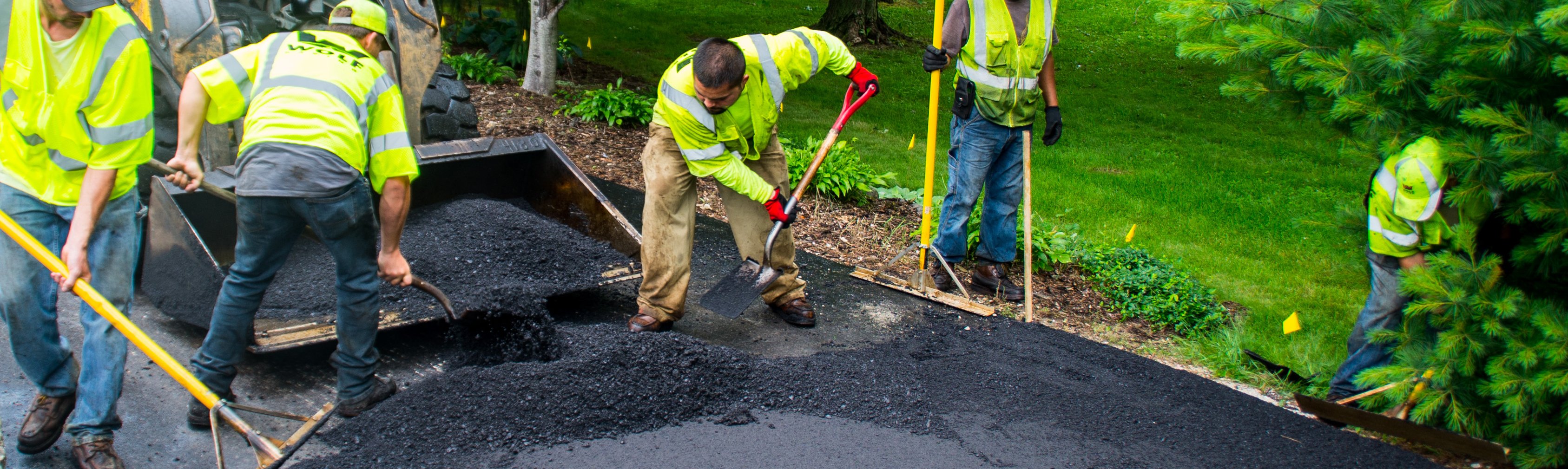In the image, several men are depicted working diligently on a task. They are positioned on a vibrant green lawn, bordered by a large tree with lush, green leaves. The lawn is dotted with small yellow flags. The scene shows the men shoveling coal from a large container onto the street. One worker stands out with a large rake, meticulously spreading the coal. All the workers are donned in yellow safety vests with reflective gray stripes. While some are focused on shoveling and raking the coal, another worker appears to be taking measurements, and one more can be seen walking back into the surrounding bushes, possibly to retrieve more equipment or check on something.